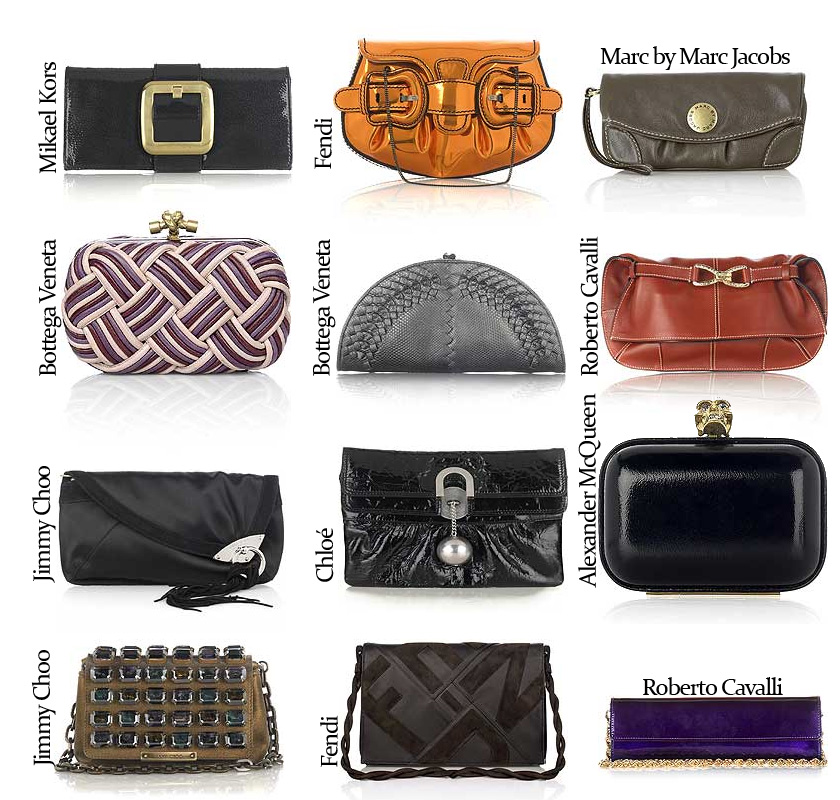This promotional image showcases 12 assorted handbags, neatly arranged in four rows and three columns against a clean white background. Each handbag is distinct in design, color, and brand, creating a captivating display of luxury and style. 

Starting from the top left:

1. **Michael Kors**: A black handbag featuring a prominent gold buckle.
2. **Bottega Veneta**: An artfully crafted bag made of braided cords in shades of purple, mauve, and pink with a gold clasp.
3. **Jimmy Choo**: A rectangular handbag wrapped in a shiny fabric with a silver fastener and delicate tassels.
4. **Jimmy Choo**: Another variant, this time a leather handbag adorned with numerous small buckles.

In the middle column:

5. **Fendi**: A vibrant orange handbag.
6. **Bottega Veneta**: A gray handbag shaped like a half-circle with a woven edge.
7. **Chloe**: A sleek black handbag highlighted by a large silver fastener.
8. **Fendi**: A black handbag featuring a distinctive textured logo sewn into the surface.

In the third column:

9. **Mark by Mark Jacobs**: A taupe handbag with a gold fastener.
10. **Roberto Cavalli**: A striking red handbag with a gold fastener.
11. **Alexander McQueen**: A black, rectangular handbag reminiscent of a CD case with a gold fastener.
12. **Roberto Cavalli**: A slender purple handbag accented by gold fringe or a strap at the bottom. 

The handbags vary in shape, style, and color, ranging from black, orange, red, pink, and purple, showcasing a range of luxurious designs and intricate detailing.